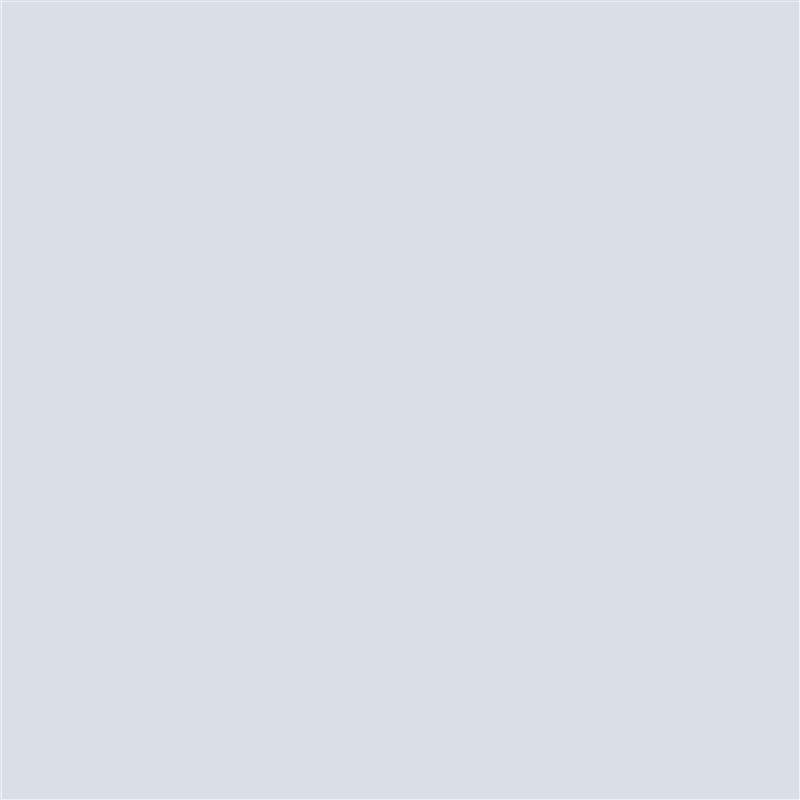The image depicts a perfectly uniform, solid gray square. The shade of gray is consistent throughout, with no variations or additional tones. There is no content or design within the square; it is entirely monochromatic. The simplicity and uniformity make it devoid of any distinguishing features or subjects. This gray square could potentially be used as a background to overlay other images or text, but in its current state, it remains a completely blank gray canvas, devoid of any additional elements or embellishments.